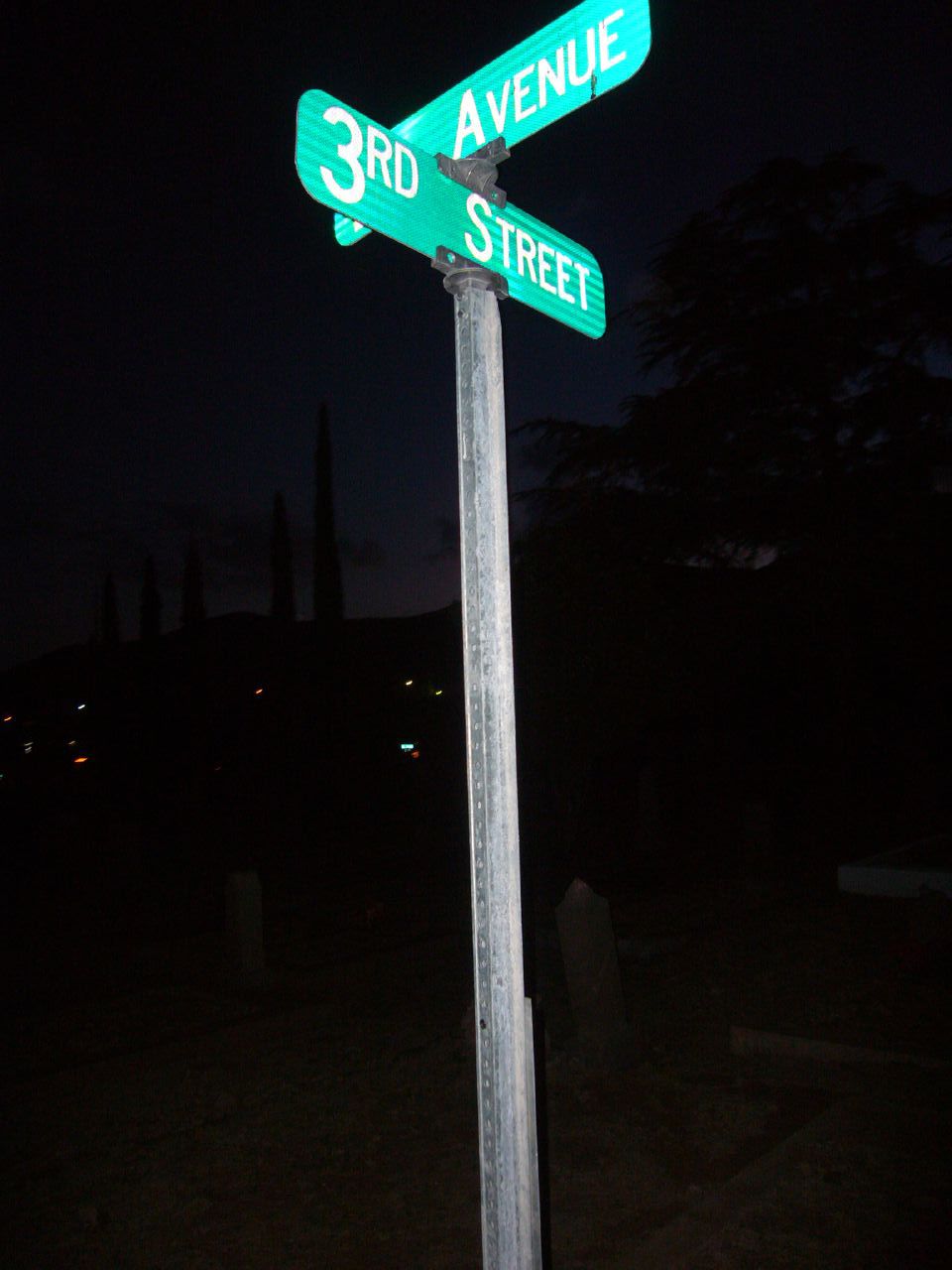This horizontally oriented nighttime photograph, flipped 90 degrees counterclockwise, features a prominently lit street sign at its center against a dark, barely discernible cityscape. The illuminated street sign, supported by a tall silver metal pole, displays two green street signs with white text. These perpendicular signs read "3rd Street" on one and partially obscured "Avenue" on the other. The background reveals only faint silhouettes of buildings and a very dim transition from sky to cityscape, further emphasizing the street sign as the focal point in this otherwise shadowy image.